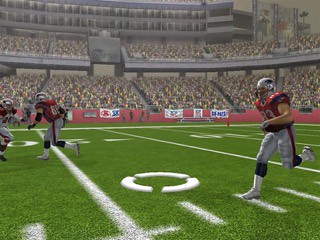This image is a slightly blurry screenshot from a football-themed video game, characterized by its vintage graphics likely from the 2000s to 2010s. At the center of the brightly green football field, distinguished by its white striping and yard markers, there's a white circular marker that presumably signifies the player's cursor. The field is populated with players clad in uniforms: gray helmets, red jerseys, and white pants with red stripes, adding to their detailed appearance.

There are three main players in this scene. On the right, one player is running leftwards towards the center marker. On the left edge, two other players are seemingly racing towards each other, running side-by-side. The stadium, bustling with spectators donned in a patterned mix of yellow and red, serves as the backdrop. Additionally, there are stairways between the bleachers and various exit points scattered around. Further detailing includes a large building in the background and a red border filled with signs and advertisements beneath the stands.